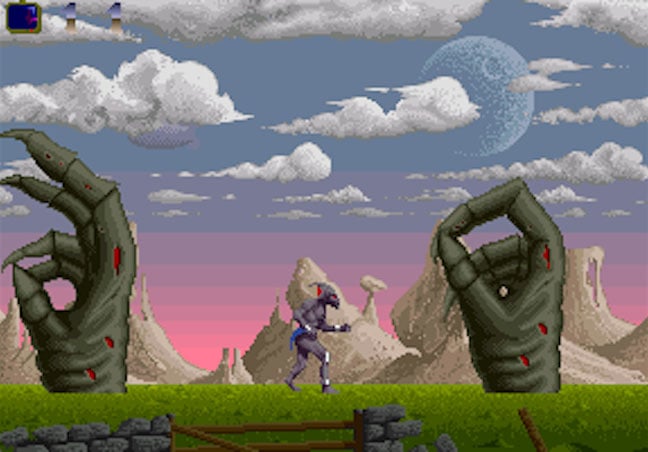This image is a screenshot from an old, retro-style pixelated video game. At the center of the scene is a humanoid character with an angular head and red eyes, wearing a blue loincloth. The figure is well-muscled and bare-chested, adorned with white wristbands and straps around his knees and ankles. He walks in a grassy field defined by a stone and wood fence, with two large, eerie hands emerging from the ground on either side of him—one hand is open and the other is closed. The hands are black with red marks that resemble injuries. The background features a dry, desert-like mountain landscape under a sky painted with hues of purple and pink from the setting sun, along with a blue moon and scattered clouds.